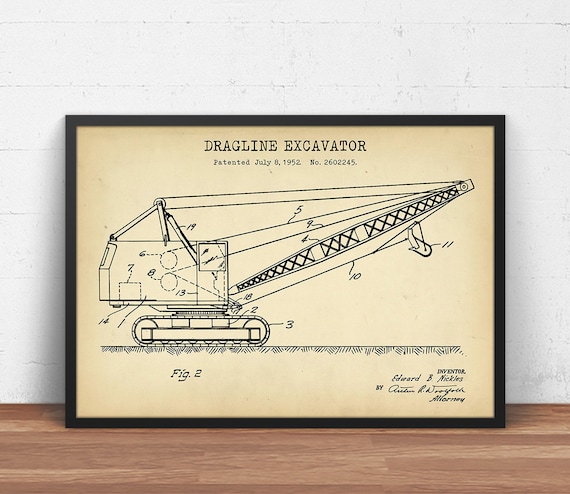The image depicts a horizontally oriented rectangular picture frame resting on a light wood-colored floor, leaning against a faintly outlined white brick wall. The black frame, which is not very wide, encloses a vintage-looking illustration of a dragline excavator, resembling a dated patent diagram. The paper of the illustration bears a slightly yellowed, aged appearance. At the top of the illustration, in large black letters, it reads "Dragline Excavator," followed by "Patented July 8th, 1952" and the patent number "2602245" in smaller text. The depicted dragline excavator, which looks like a crane with tractor-like wheels, extends to the right side of the image, with labeled ground depiction beneath it. Below the illustration, the caption "Figure 2" is visible, along with various cursive signatures of the inventors on the bottom right corner.